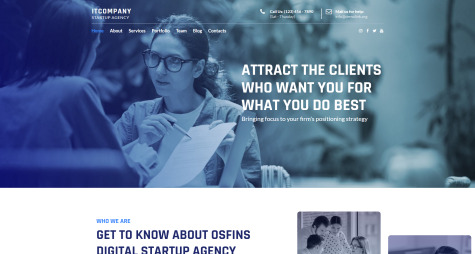In the background of the image, a cool blue overcast sets the scene. In the foreground, a woman with glasses and her hair neatly pulled back into a ponytail is featured. She holds a piece of paper in one hand, and with the other hand, she points to the document using a pen. Across from her, the back of another woman's body is visible, with only the rear view of her long hair and long-sleeved t-shirt in sight.

At the top of the image, white text reads, "IT company, attract the clients who want you for what you do best." A telephone symbol accompanied by faint, small text is also positioned at the top. Below, a blue section with text introduces "OSFINS," a digital startup agency, inviting viewers to know more about "who they are."

To the right, a small square contains an image of a family gathered around a laptop, presumably in an informational setting. The family includes a mother, a father, a teenage daughter, and likely a teenage son, all focused on the screen before them.